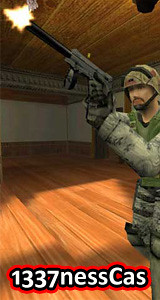In this dynamic and vividly illustrated image, reminiscent of a scene from a military or shooting video game, we observe a soldier clad in detailed military camo attire. Only the right half of his figure is visible as he emerges from the right-hand side of the frame. The soldier is actively engaged in combat, aiming a pistol fitted with a large silencer towards the top-left corner of the image. His head is protected by a sturdy helmet, indicating his readiness for battle.

The setting appears to be an indoor, cartoony environment, characterized by a wooden floor, white walls, and a wooden ceiling. Adding to the action-packed atmosphere, a small explosion graphic is depicted at the point where the soldier's pistol is aimed, suggesting he has just fired a shot. Below this intense scene, the player's gamer tag "1337 NESSCAS" is prominently displayed, grounding the image firmly in the realm of interactive entertainment.